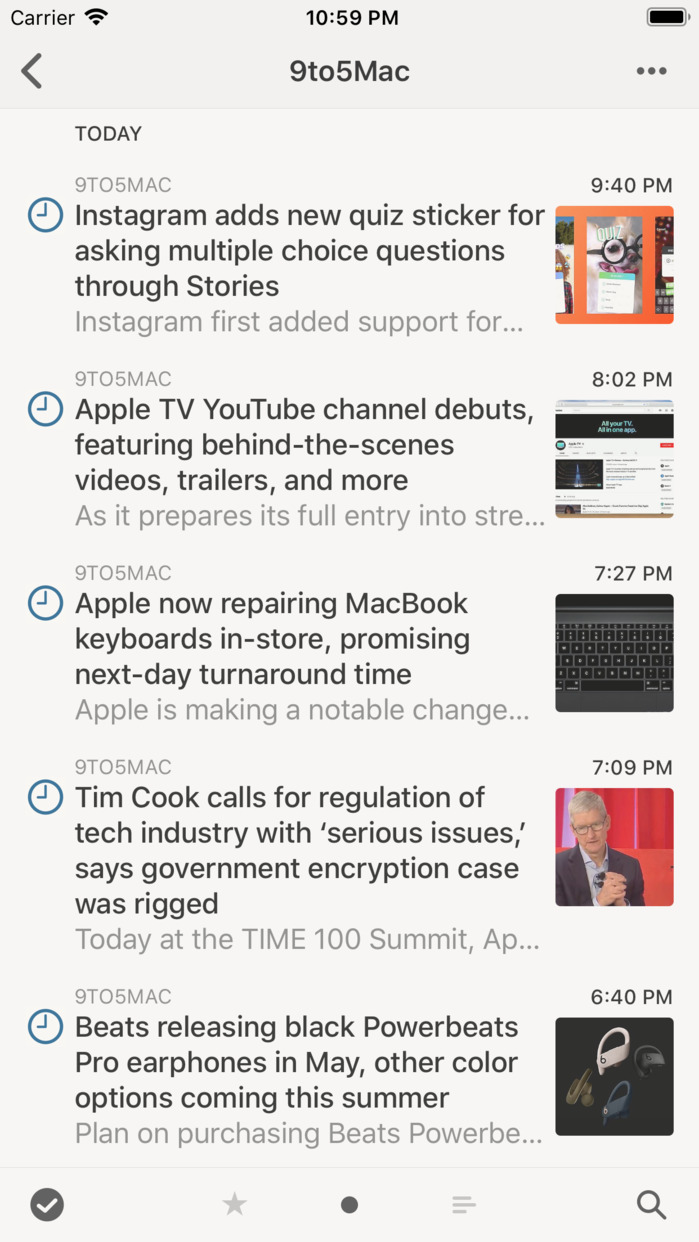This screenshot captures notifications from the 9to5Mac app on a smartphone, showcasing five recent updates from the iOS-focused news outlet. Each notification features a headline, a brief excerpt from the article, a corresponding image, and the time it was posted. From top to bottom, the notifications detail various news stories, such as an announcement about Instagram adding a new quiz sticker for multiple-choice questions in stories, posted at 9:40 AM. The other articles were posted at 8:02 AM, 7:27 PM, and 7:09 PM, ensuring fresh content is available nearly every half hour. The top of the screenshot indicates these updates are from today, providing readers with timely and relevant information. Each notification is visually supported by a small image to the right, enhancing the user's browsing experience and helping them decide which article to read next.